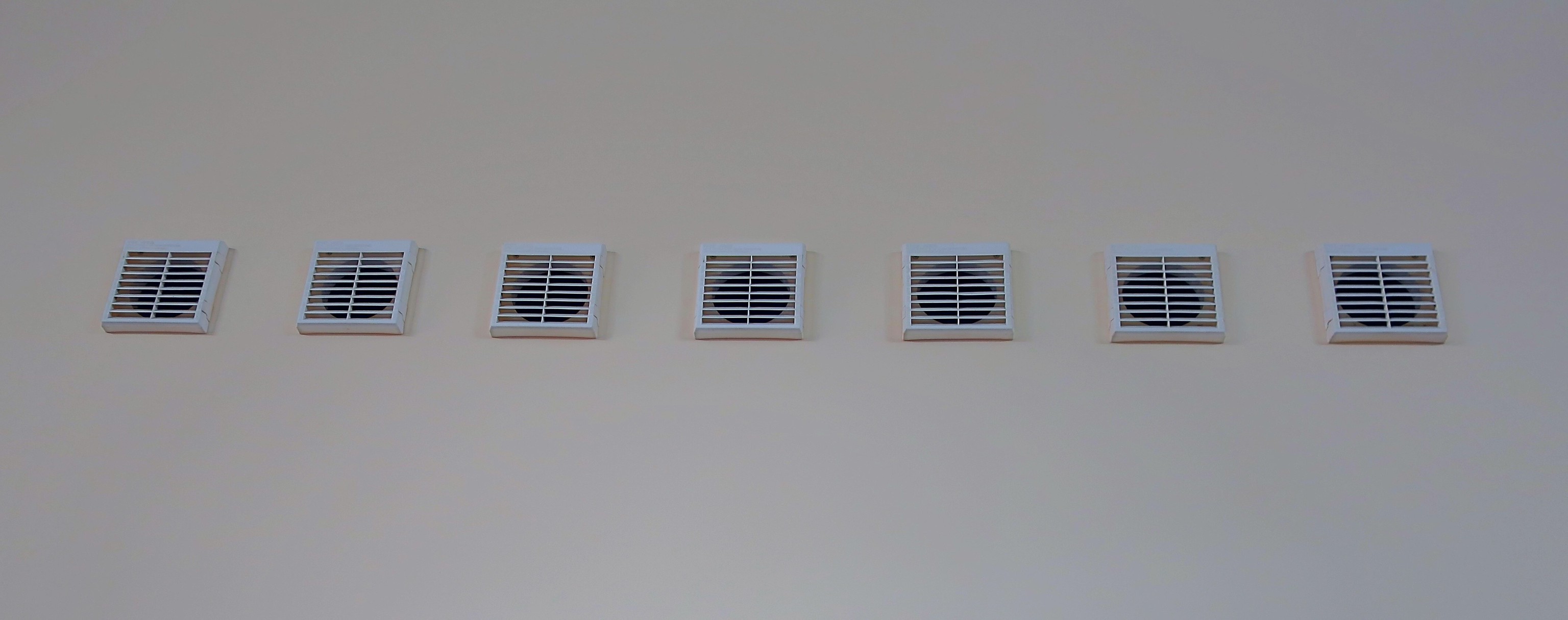This image shows seven square vents aligned horizontally in a symmetrical row against a cream-colored wall, possibly on the exterior of a building. Each vent features horizontal slats with a central seam, revealing a dark circle behind the slats, suggesting they cover a fan or exhaust mechanism. The vents are white, contrasting against the slightly off-white background, and their uniform placement creates a harmonious and orderly pattern. The outer edges of the vents are thicker, adding to their distinct appearance. The overall scene is detailed and precise, highlighting the industrial design of the vents against a subtly shaded wall.